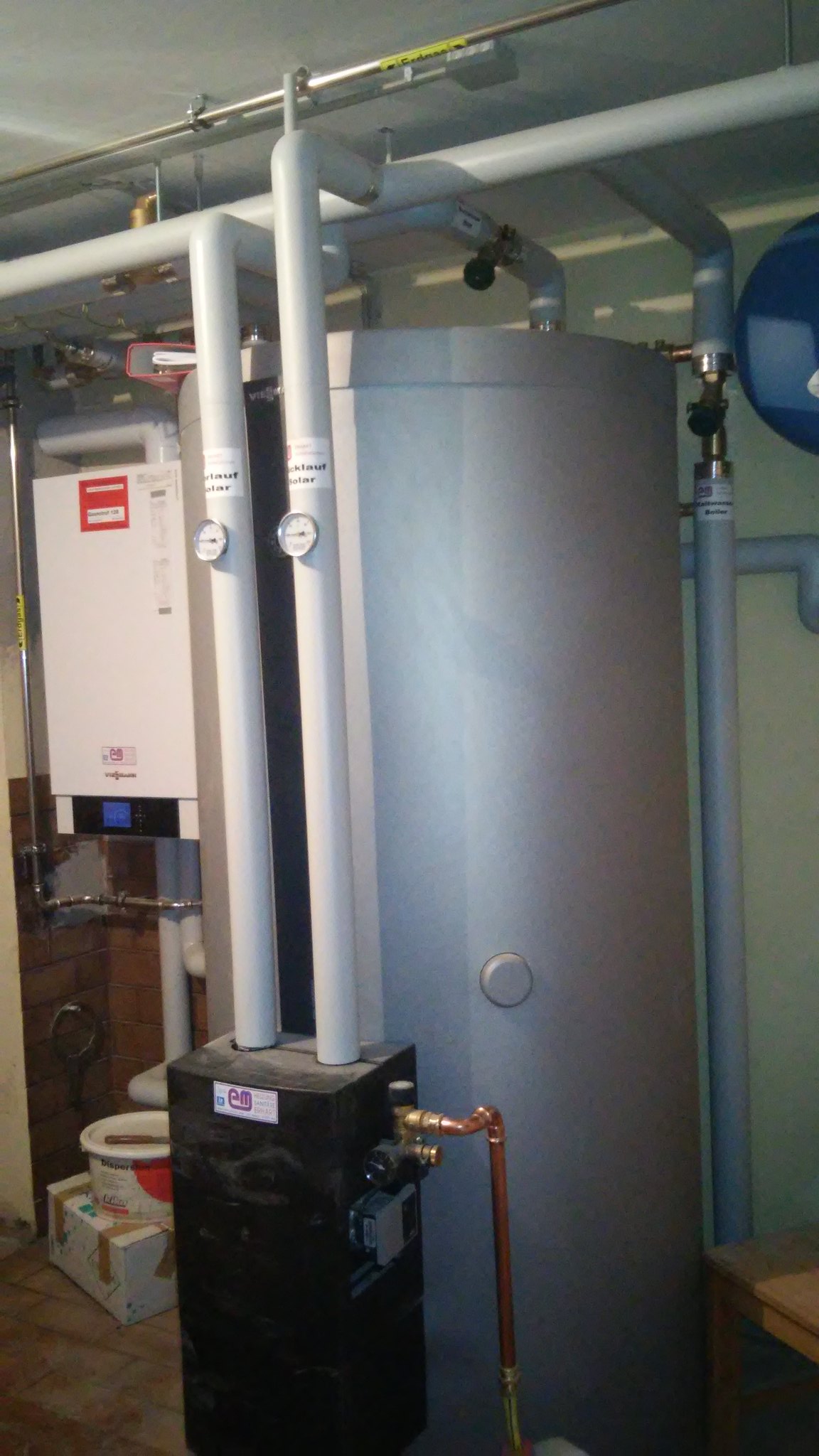This color photograph appears to be taken inside a room, possibly a basement or an industrial space, characterized by light-colored walls and a white ceiling. The focal point of the image is a large, gray-colored cylindrical water heater, prominently placed among a complex network of water pipes. Several white pipes extend the length of the room, connecting to a horizontal metallic-colored pipe and further branching off in various directions. Two of these pipes descend into a shiny, black rectangular box mounted to the wall, featuring a copper pipe on its right-hand side. This box appears to be some sort of control system, possibly for regulating water flow. In the background, another white box, likely an electric unit or a coolant system, is visible with additional water lines connected to it. The overall setting has an organized yet industrial feel, with numerous pipes running throughout the room, suggesting a space designed for significant water handling or possibly a specialized function like a chemistry lab. Various items can be seen on the floor, adding to the functional and utilitarian atmosphere of the room.